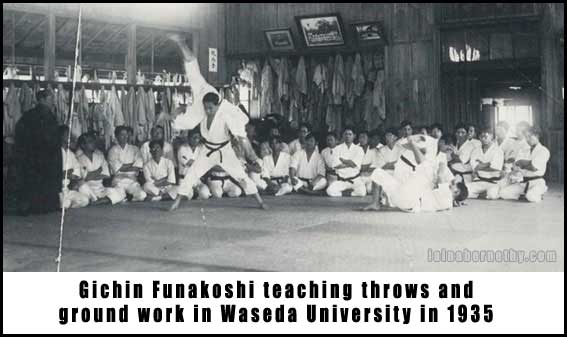The black and white photograph captures a significant moment from 1935 at Waseda University, where Gichin Funakoshi, renowned as the founder of modern Karate, is demonstrating throws and groundwork techniques. At the heart of the image, Funakoshi is shown executing a throw, hoisting a practitioner over his shoulder. Surrounding him, approximately 20 to 30 male students, dressed in traditional white karate uniforms with dark belts, are seated on the floor, attentively observing the demonstration. The setting appears to be a large wooden dojo, its background adorned with hanging robes and a few framed pictures. Sunlight softly streams in through the door, illuminating the focused expressions of the students and the historic martial arts instruction taking place.